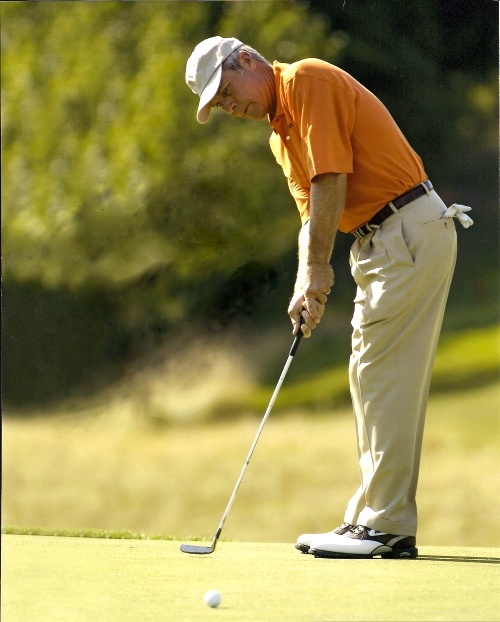The photograph captures an older man engaged in a golf game on a sunny day. He is positioned in the center of the image, standing on a well-manicured, flat grassy area. His body is turned slightly to the left as he bends over in the posture of having just executed a putt. In his hands, he holds a simple silver golf club with a black grip. The golf ball, recently struck, is visible on the green near the bottom of the image. The man sports an orange collared polo shirt, buttoned up, and a white or beige cap atop his gray hair. He is dressed in beige slacks with a dark brown or black belt, and a pair of white gloves protrudes from his back pocket. His footwear consists of white Nike shoes with gray accents. The background is a blurry mix of trees and grassland, emphasizing the golfer and the immediate green while suggesting a lush, vibrant setting typical of a well-maintained golf course.